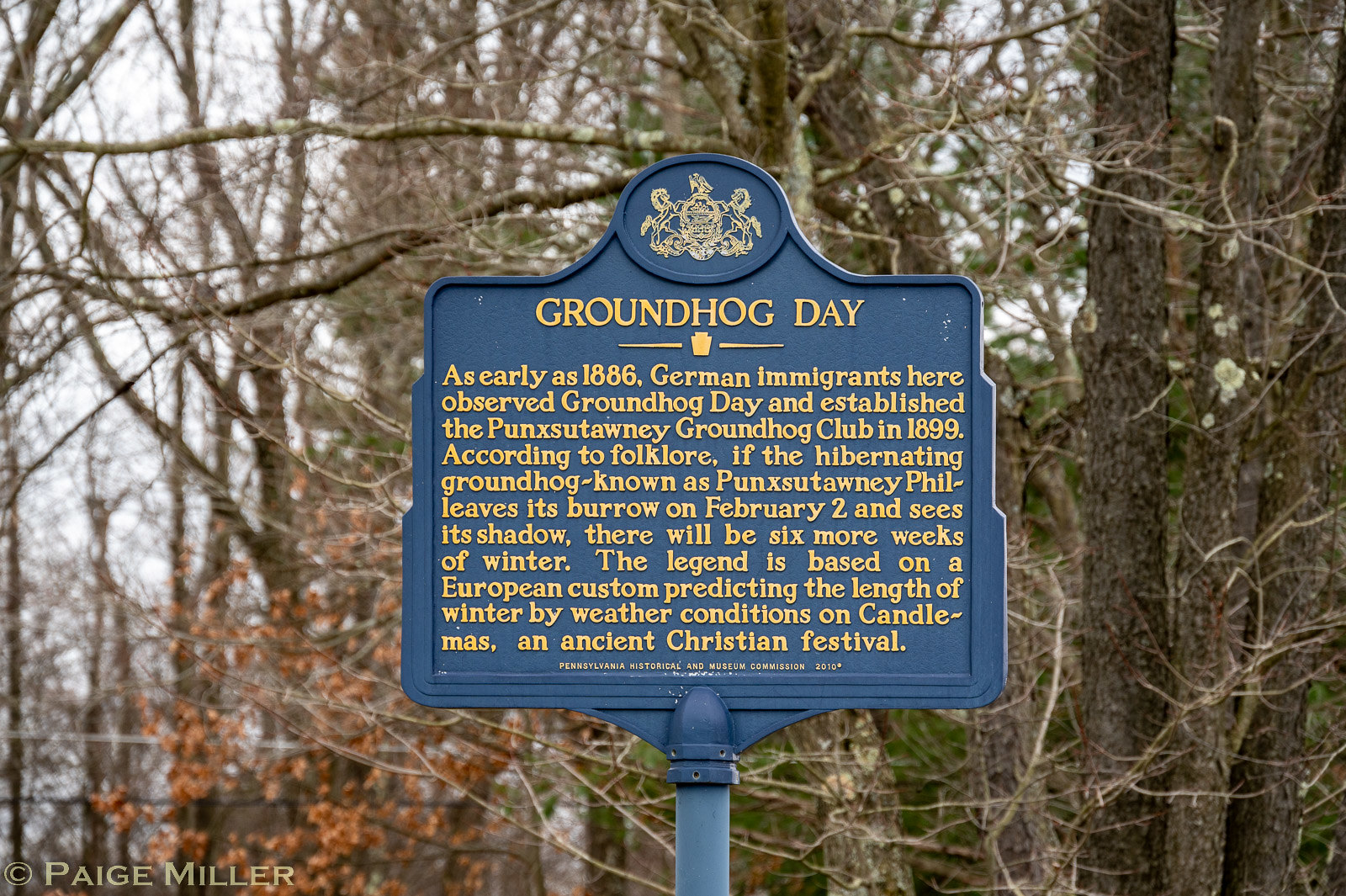The image features a blue metal sign standing on a matching blue pole, placed in front of a forest of dry, mostly leafless trees. The oval-shaped sign has a rounded top that includes an insignia, and beneath it, in prominent yellow-green letters, are the words "Groundhog Day." The text on the sign, also in yellow, reads: "As early as 1886, German immigrants here observed Groundhog Day and established the Punxsutawney Groundhog Club in 1899. According to folklore, if the hibernating groundhog known as Punxsutawney Phil leaves its burrow on February 2nd and sees its shadow, there will be six more weeks of winter. The legend is based on a European custom predicting the length of winter by weather conditions on Candlemas, an ancient Christian festival." The sign stands amid a wild-looking forest with some dead leaves scattered, giving a desolate feel to the surroundings.